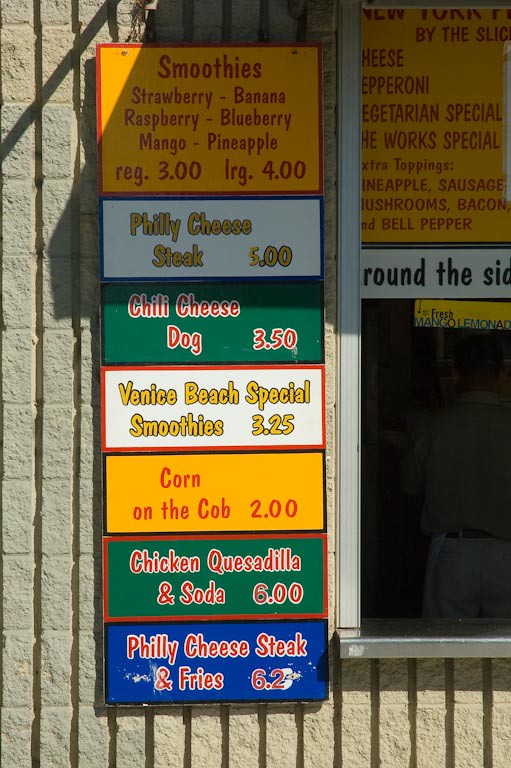This outdoor photograph showcases a concrete wall segmented to resemble individual bricks, adorned with several vibrant signs advertising various food and drink items. The first sign is orange with playful red handwriting, listing smoothie flavors including strawberry, banana, raspberry, blueberry, mango, and pineapple, with prices of $3.00 for a regular size and $4.00 for a large. Next, a white sign with bold yellow lettering and black outline advertises a Philly cheesesteak for $5.00. The unique detail of gold for the number "5" and black-outlined zeros suggests a recent price update.

A green-background sign with red text follows, offering a chili cheese dog for $3.50. Adjacent is a white sign with gold lettering outlined in black, promoting a Venice Beach special smoothie for $3.25. Below, a golden sign with red text advertises corn on the cob for $2.00. Continuing down the list, a green sign with red writing offers a chicken quesadilla and soda for $6.00. At the bottom, a blue sign, partially worn, advertises a Philly cheesesteak and fries for $6.2X, with the last digit obscured.

To the right of these signs, an open window reveals a slightly darkened interior with a person only partially visible, possibly wearing a button-down shirt, white pants, a dark belt, and an apron. Above the window, an additional sign is partially cut off, but the legible text includes items like "New York something," "buy the slice," "cheese," "pepperoni," "vegetarian special," and varied toppings including pineapple, sausage, mushrooms, bacon, and bell pepper arranged around an obscured word. The bright daylight outside contrasts with the dimmer interior, capturing a bustling yet inviting outdoor food stand ambiance.